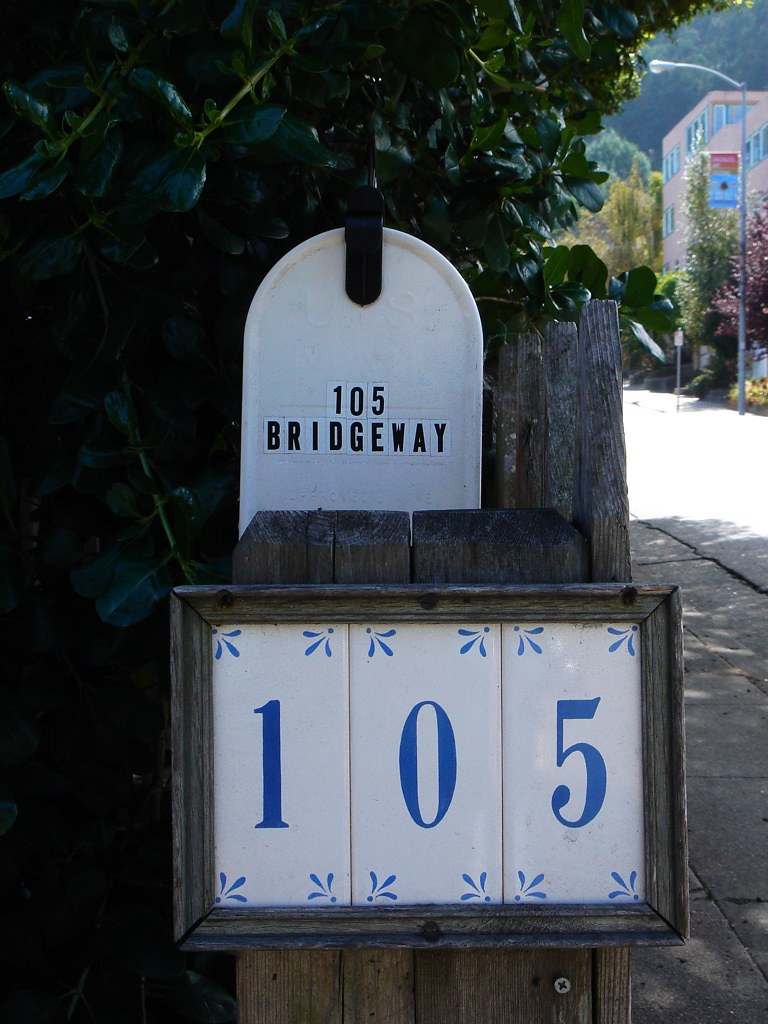The image captures a white mailbox prominently centered in the upper half of the frame, mounted on a vertical plank fence. The mailbox, featuring a black handle, displays the letters "Bridgeway" and the numbers "105." Below the mailbox door is a large sign framed in dark grayish-brown wood, featuring ceramic numbers "105" in blue. Surrounding the mailbox, there is lush green shrubbery visible at the top of the frame. To the right, the view extends to a street with a distant pink and blue three-story building and a light post in front of it.